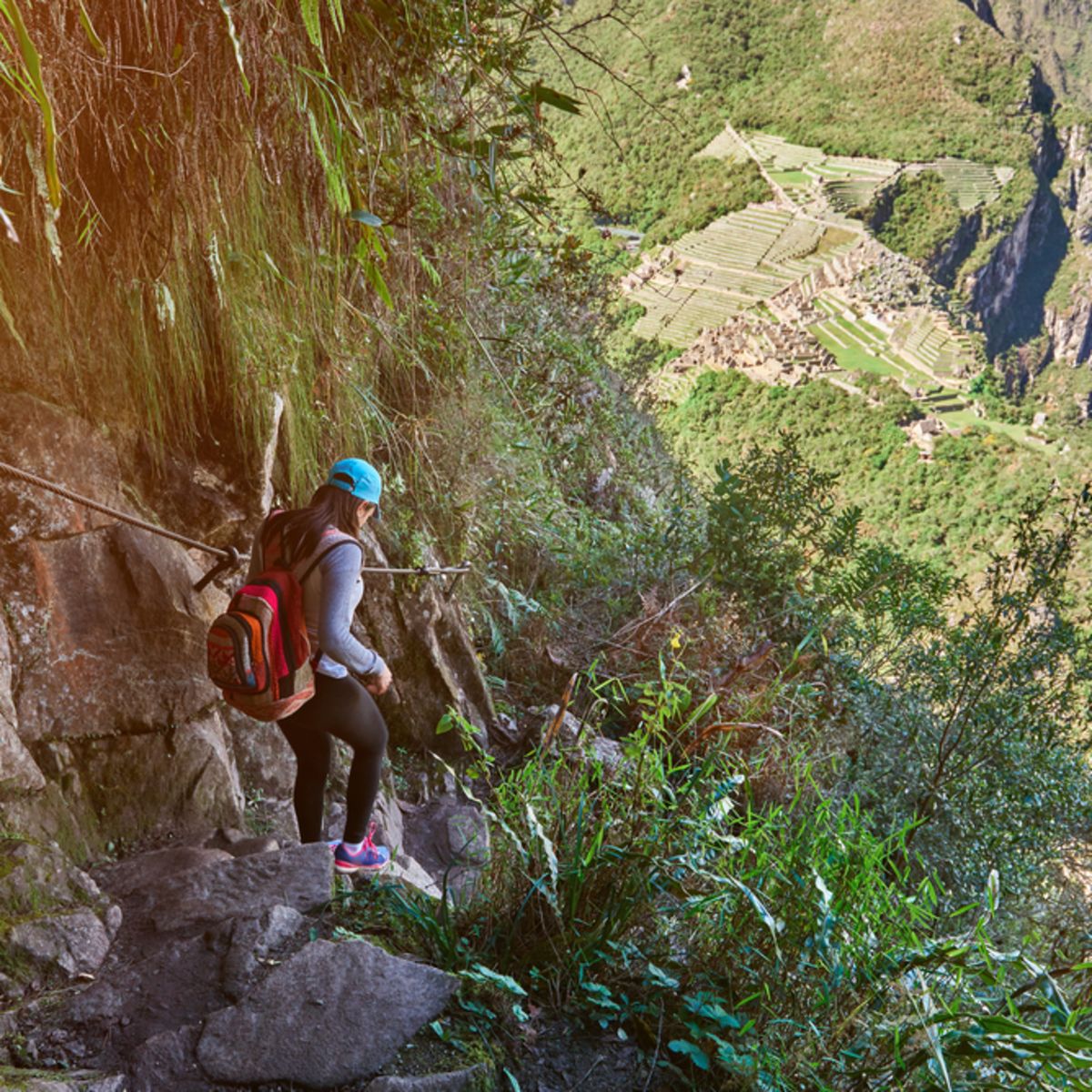In the vivid image, a woman with long brown hair is captured hiking in a mountainous and rocky terrain. She is donned in a blue cap, a light gray long-sleeved shirt, black leggings, and colorful hiking shoes in shades of pink and blue. A striking red backpack is strapped to her back, and a harness attached to a rope is visible, indicating a potentially challenging hike. She is navigating a rocky path at the top of a steep cliff, with the ground level appearing to be thousands of feet below, filled with dense greenery and trees. The landscape around her is a mix of rocky formations and lush vegetation, with shadows cast by the terrain in certain areas while other parts are bathed in sunlight. The image captures the blend of natural beauty and the adventurous spirit of the hiker amidst the rugged, green-laden mountain range.